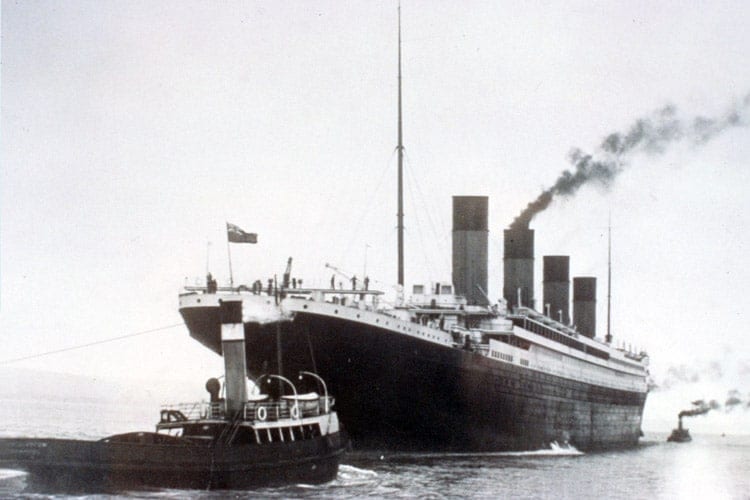This vintage black-and-white photograph captures the grandeur of a massive steamship, evocative of the Titanic, on a calm ocean during daylight. The enormous ship dominates the scene with four towering smokestacks, the second one billowing black smoke, and a distinctive flag perched at the front. The hull is dark, contrasting with the lighter upper decks, and the ship appears well-populated with visible figures on deck. Two tugboats, positioned at the front left and rear of the ship, assist in maneuvering. The tugboat in the foreground is small, white-and-black, and connected to the steamship by a rope. Both tugboats have smokestacks emitting smoke, adding to the dynamic yet serene atmosphere of the image. The sky is cloudy, creating a moody backdrop to this historical maritime scene.